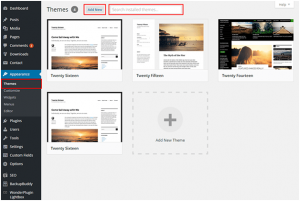This screenshot captures the 'Themes' section within the WordPress admin dashboard, specifically located under the 'Appearance' tab. Dominating the upper portion of the page is a prominently highlighted 'Add New' button, inviting users to explore and install new themes. Adjacent to this button, a search bar facilitates the search for specific themes for installation. Below, the available themes are displayed in a grid format, featuring default WordPress themes like 'Twenty Sixteen,' 'Twenty Fifteen,' 'Twenty Fourteen,' and 'Twenty Seventeen,' along with options to add new themes.

On the left-hand side of the dashboard, the sidebar navigation menu is visible, listing all the main sections: Dashboard, Posts, Media, Pages, Comments, Appearance (with sub-items Themes, Customize, Widgets, Menu, Header, and Background), Plugins, Users, Tools, and Settings. The overall design of the dashboard is clean and organized, aimed at helping users efficiently manage and customize their WordPress sites by selecting and modifying themes to suit their needs. The visual layout emphasizes ease of navigation and accessibility, supporting users in achieving their website customization goals.